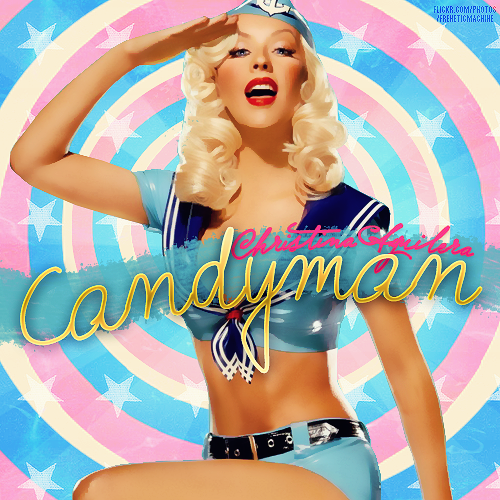This square-format color illustration features Christina Aguilera styled in retro, vintage fashion. She is depicted in a sailor-inspired outfit with a blue military-style cap adorned with an anchor, platinum blonde curls, and vibrant blue eyes. Christina wears a crop halter top that cuts off below the chest, revealing her midriff, with a dark blue scarf tied in the front and short light blue hot pants held by a dark blue leather belt. She strikes a salute with her right hand while her head tilts back slightly, and her left leg is lifted parallel to the frame of the image. Christina sports bright red lipstick, enhancing her classic look.

The background resembles a multi-colored bullseye in hues of pink, white, light blue, and traces of yellow, with white stars scattered across it. The center of the image is marked with a curved blue stripe, displaying "Candyman" in yellow, handwritten-style letters, and above in bright pink letters, it reads "Christina Aguilera." This artistic illustration has an overall stylized, retro effect, blending the charm of vintage aesthetics with a modern pop-art vibe.